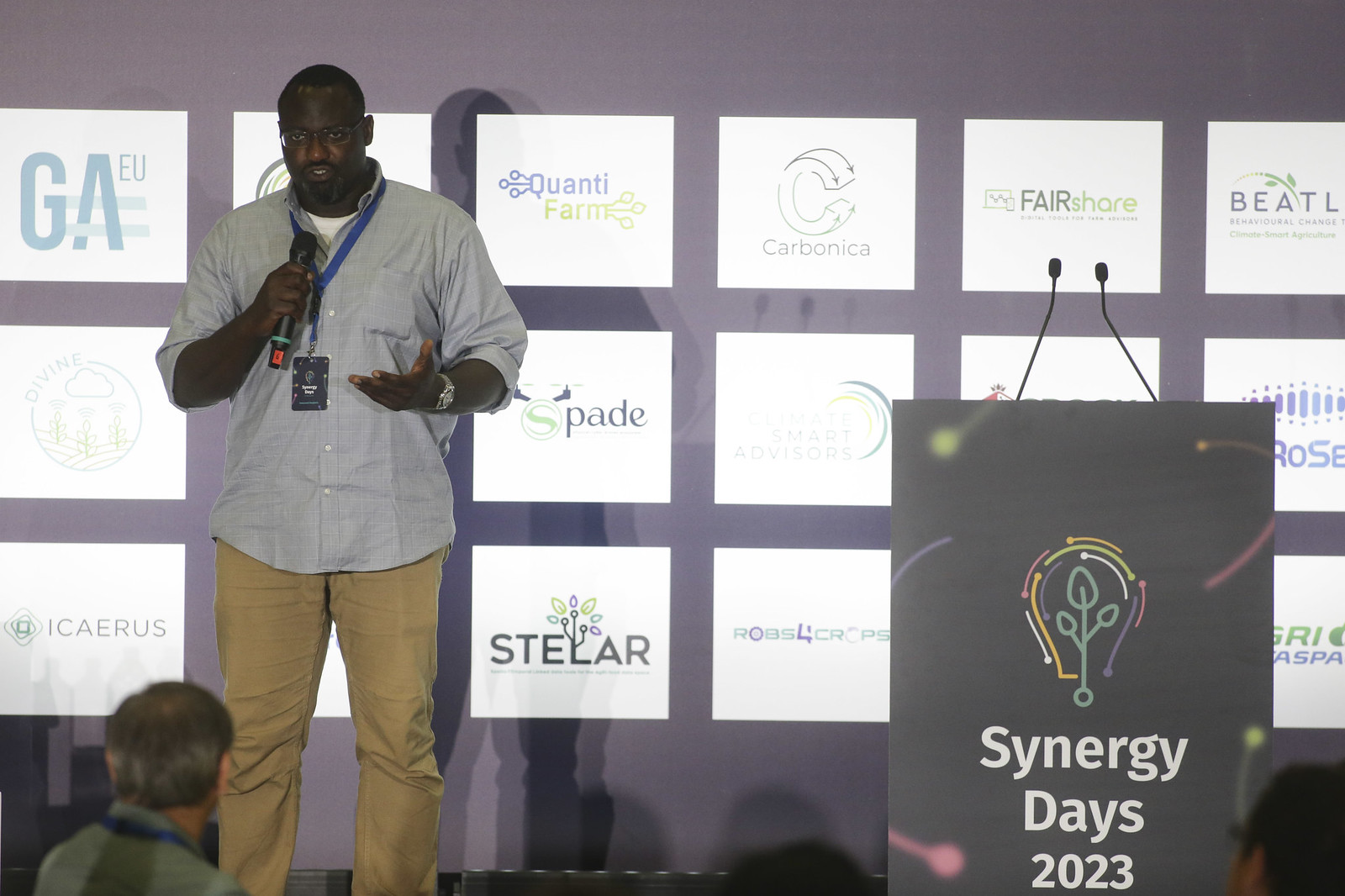The photograph captures an engaging moment at an event, prominently featuring an African-American man who appears to be speaking to a crowd. Dressed in a sky-blue button-up shirt with rolled-up sleeves and khaki, chino-style pants, he holds a microphone in his right hand while gesturing with his left. The man, who also wears a silver watch on his left wrist, stands to the left of a podium, which features a sign reading "Synergy Days 2023" and has two additional microphones attached to it. 

The backdrop is a striking contrast of a black wall adorned with an array of white squares, each displaying different company logos, including G-A-E-U, Quanti Farm, Carbonica, Fair Share, Beetle, Spade, Stellar, and Icarus. In the lower right corner of the image, part of another man’s head—gray-haired and attentive—can be seen, along with the ear and hair of yet another person, both indicating the speaker's audience. The colorful mix of logos and the varied color palette, including shades of blue, green, yellow, orange, and light brown, add vibrancy to the scene.